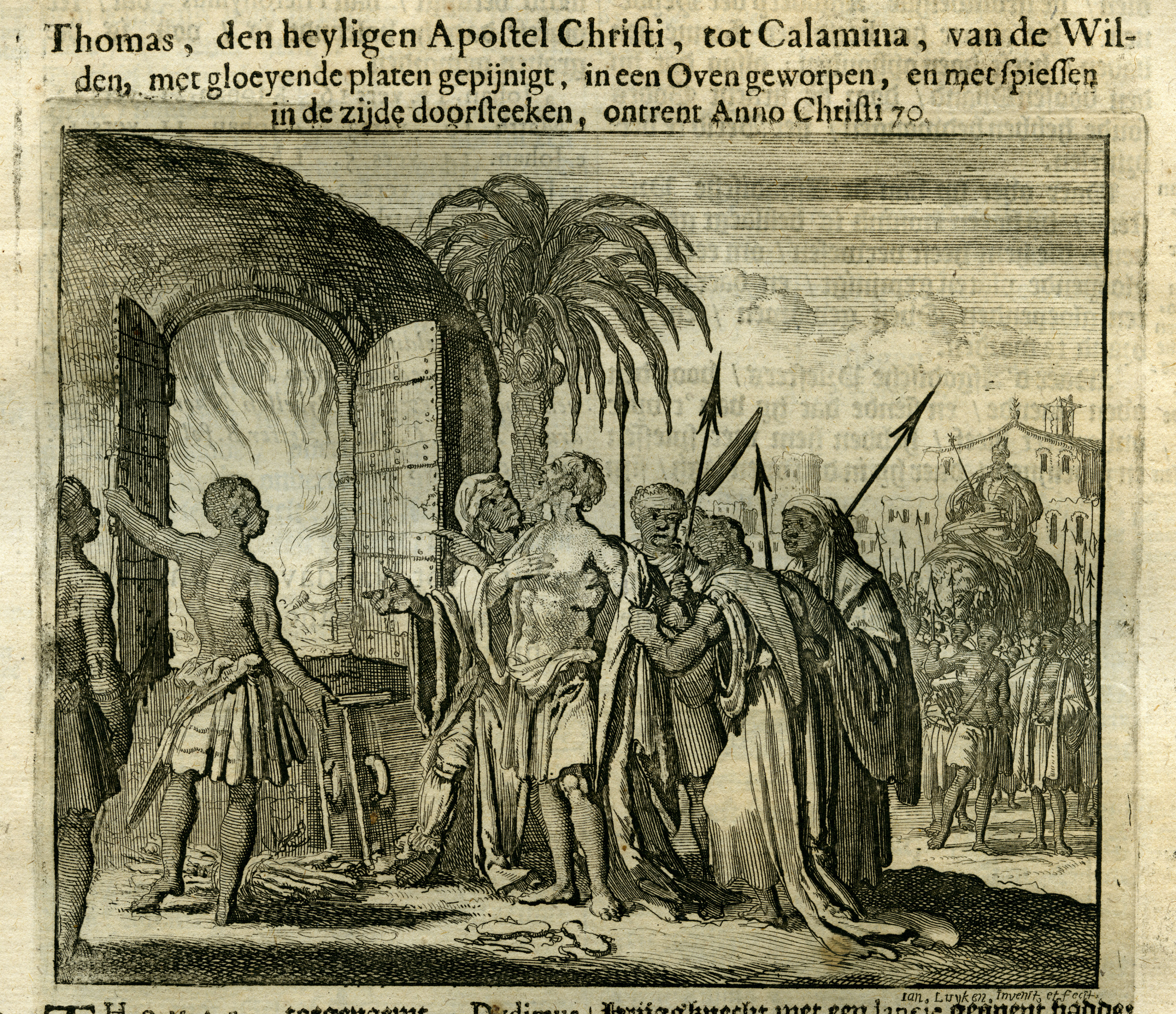The black and white image appears to be an old engraving or drawing, possibly dating back centuries. It depicts a dramatic scene involving a man who is almost naked, clad only in a cloth skirt, being held captive by several other men. The captive man is looking up towards the upper left of the image, appearing distressed. Around him, several figures wield spears, some restraining him with angry expressions. To the left, an individual seems to be explaining something to the captive, gesturing with his hand.

In the lower left, a Black man is depicted holding the door of an oven or large hut, which has visible flames inside, and he is looking at the captive man. Another Black man in a skirt is nearby observing the situation. In the background, there is a palm tree, an Arabic-style building, and a large animal, likely an elephant, ridden by another figure holding a spear.

At the top of the image, text in a foreign language is seen, with the discernible words "Thomas den Helgen Apoftel Griffithi." The scene is crowded, with about ten people in the background, adding to the tension and intensity of the scene. The artwork, marked by its intricate detailing, reflects the style of old Dutch drawings.